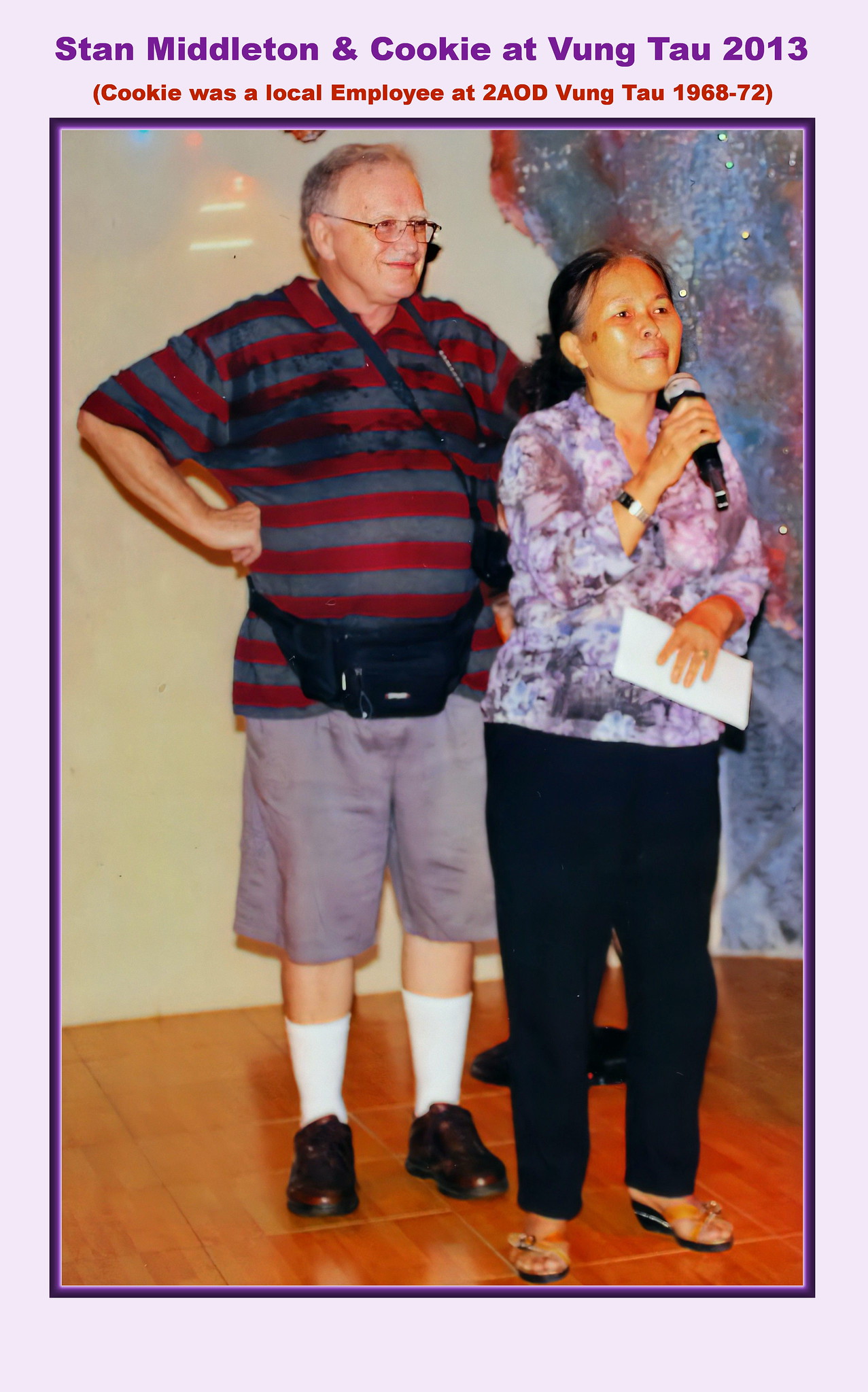This vertically aligned rectangular picture has an older appearance. It features a light gray border with a dark purple trim around the internal image. At the top, purple letters read "Stan Middleton and Cookie at Vung Tau 2013," and below that, in red parentheses, it says "Cookie was a local employee at 2AOD Vung Tau 1968-72." 

The image captures a man and a woman standing, seemingly in the midst of a karaoke session, on a brown brick-shaped floor. The man, wearing a horizontally striped red and gray polo shirt, has a black bag slung around his shoulder resting at his waist. He is dressed in gray shorts, white crew socks, and black shoes. He stands slightly behind the woman, who has darker skin, grayish-black hair, and is clad in a purple patterned top, black pants, and brown sandals. She holds a microphone in her right hand and an envelope or folded sheet of paper in her left hand.